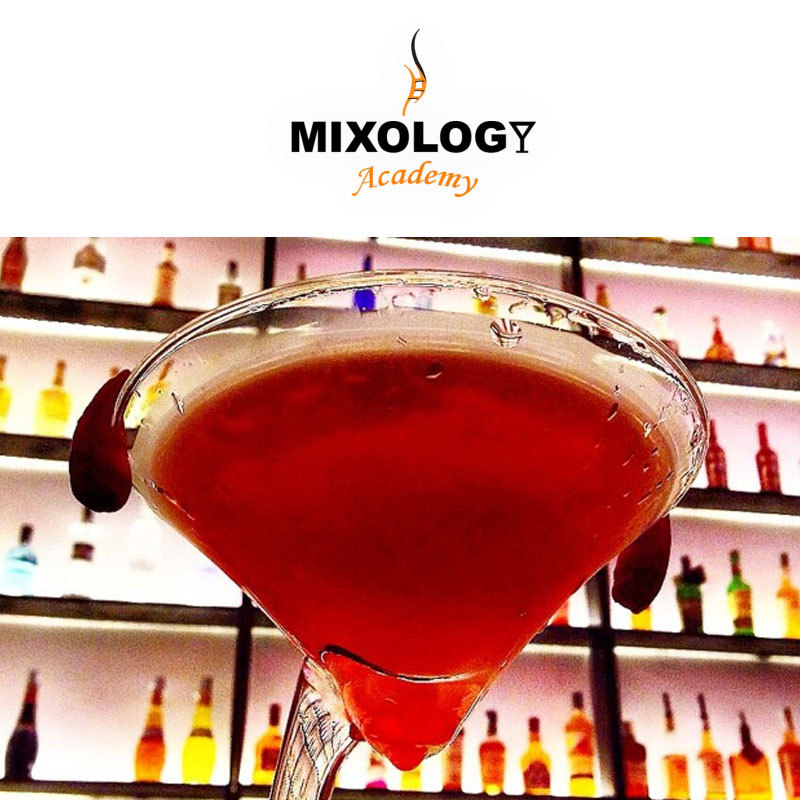This detailed image presents the "Mixology Academy" logo prominently at the top. The word "Mixology" is in bold black letters, with the 'Y' designed as a cocktail cup outline, and "Academy" is in dark yellow letters. Above the text is a small flame graphic. Below the logo is a striking photograph of a cocktail in a triangular-shaped, martini-like glass. The drink is a vibrant red and fills the glass, which has a pointed stem extending out of the frame. Water droplets speckle the glass, suggesting it's freshly served. Hanging from the glass is a red garnish, likely fruit. The backdrop features a well-lit bar with multiple shelves of liquor bottles. The shelves, dark brown, are backlit with pink and white lighting, creating a bright, colorful display. The bottles range in hue with more yellow or amber tones on the bottom shelf. The lighting beneath the shelves gives the entire scene a glowing, upscale ambiance.